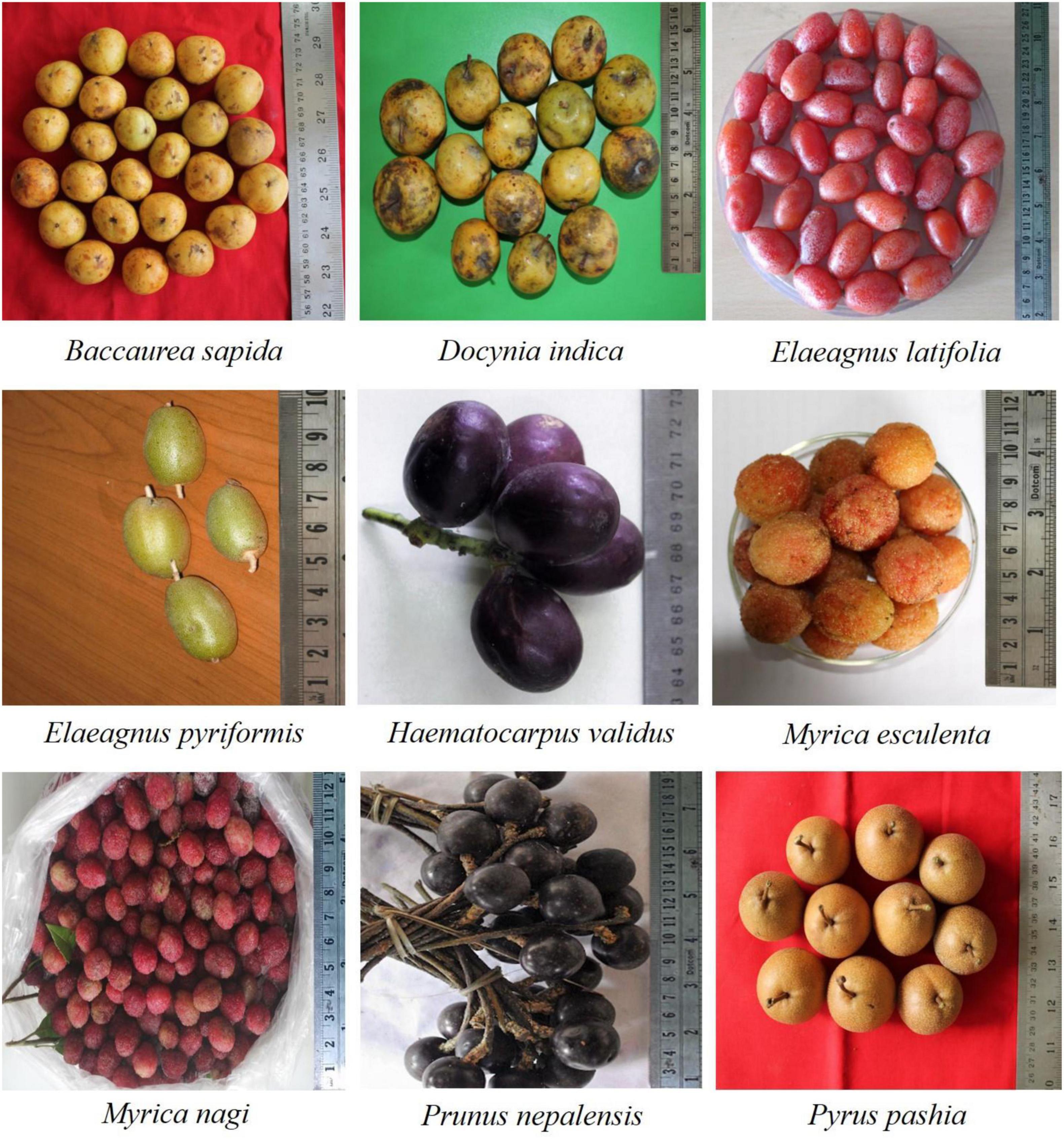This vibrant poster showcases a collection of nine distinct types of berries and fruits, each clearly displayed in individual panels arranged in three rows and three columns. Each fruit is labeled with its Latin name beneath the image, enhancing the educational value. The top left panel features light brown berries on a red background labeled "Bacchoria sapita." Next to it, on a green background, are what appear to be potato-like "Docinia indica." Completing the top row is the "Legnus latifolia," red berries set against a light gray background.

The middle row continues with "Legnus piriformis," showing four green olive-like fruits on a wooden table. Adjacent are five black olive-looking berries on a twig, labeled "Haematocarpus volitis." The final image of this row is a small glass bowl filled with orange and yellow berries referred to as "Myrica esculenta."

In the bottom row, the first image to the left is an open plastic bag containing red berries, identified as "Myrica neige." Beside it, there are two bundles of what could be plums on twigs, named "Prunus nepalensis." The final panel on the bottom right showcases nine fruits that resemble kiwis, labeled "Pyrus paschia." Each image includes a ruler to accurately display the size of the fruits, contributing to the visual appeal and informational content of the poster.